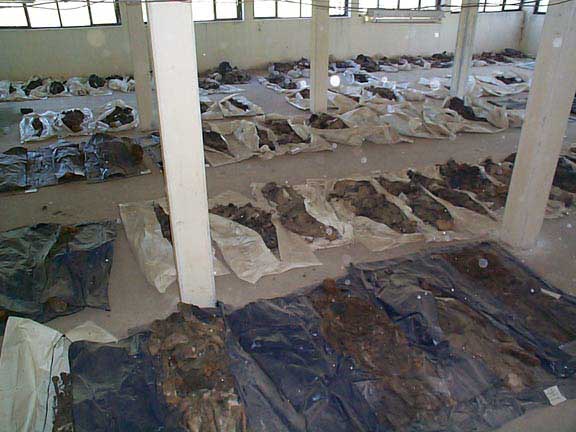The photograph captures the stark interior of a large, white-walled cement room, possibly a cellar or old warehouse. In the center of this eerily pristine space, rows of white square support columns stretch to the ceiling, framing the room's setup. The back wall is lined with a series of narrow windows, letting in minimal light that barely illuminates the scene.

Dominating the floor are orderly rows of plastic tarps: blue in the front, transitioning to white further back. Each tarp bears long, dark brown objects resembling decaying bodies or mummified remains. These shapes lack distinct features, appearing as amorphous, muddy globs lying atop the tarps. The arrangement suggests a macabre display, evoking images of exhumed, unrecognizable corpses. The overall atmosphere is chilling, with the contrast of the room’s clinical whiteness against the disturbing, cluttered mound of potential human remains.